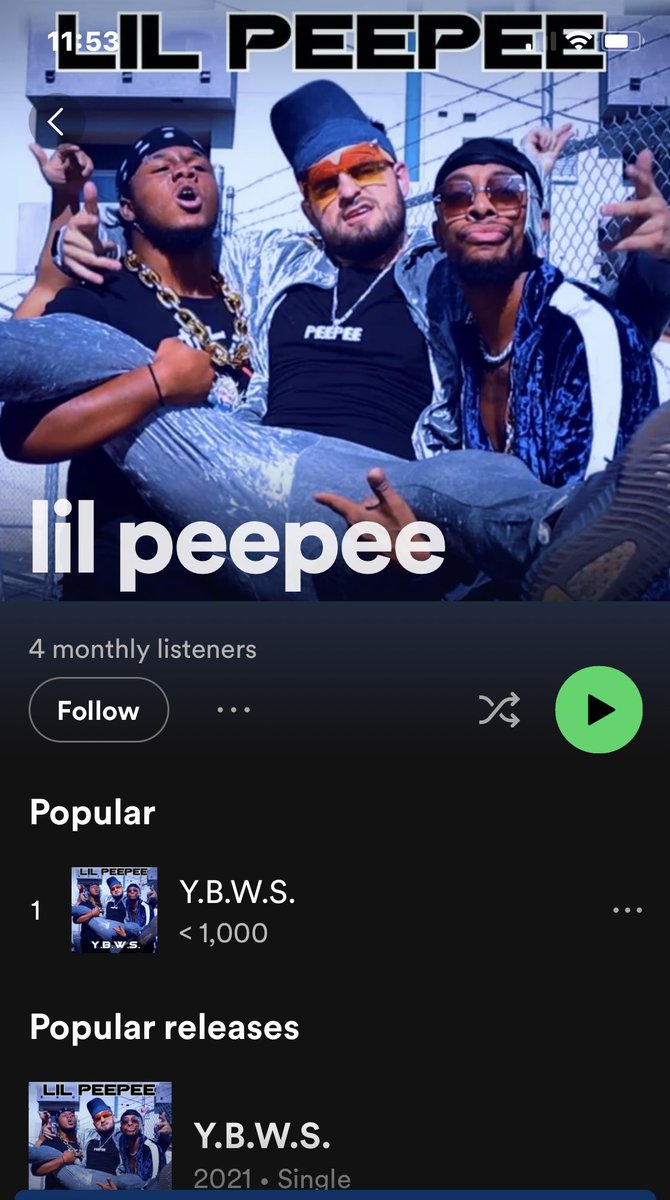The image shows a screenshot taken from a smartphone displaying a photo of a music group possibly named "Lil Peepee." In the picture, three men are posing for the camera, smiling. 

The first individual, who is African American, wears a thick chain around his neck and has a bandana over his head. He stands next to a Caucasian man wearing a hat and orange sunglasses, who also has a small chain around his neck and a shirt that says "Peepee." He sports a light mustache and beard.

Next to them is another African American man wearing large sunglasses and a hooded sweatshirt with a distinct white stripe running down the arm. He is making a peace sign with his hand. 

The screen also shows UI elements with a play button and sections for "Popular" and "Popular Releases."